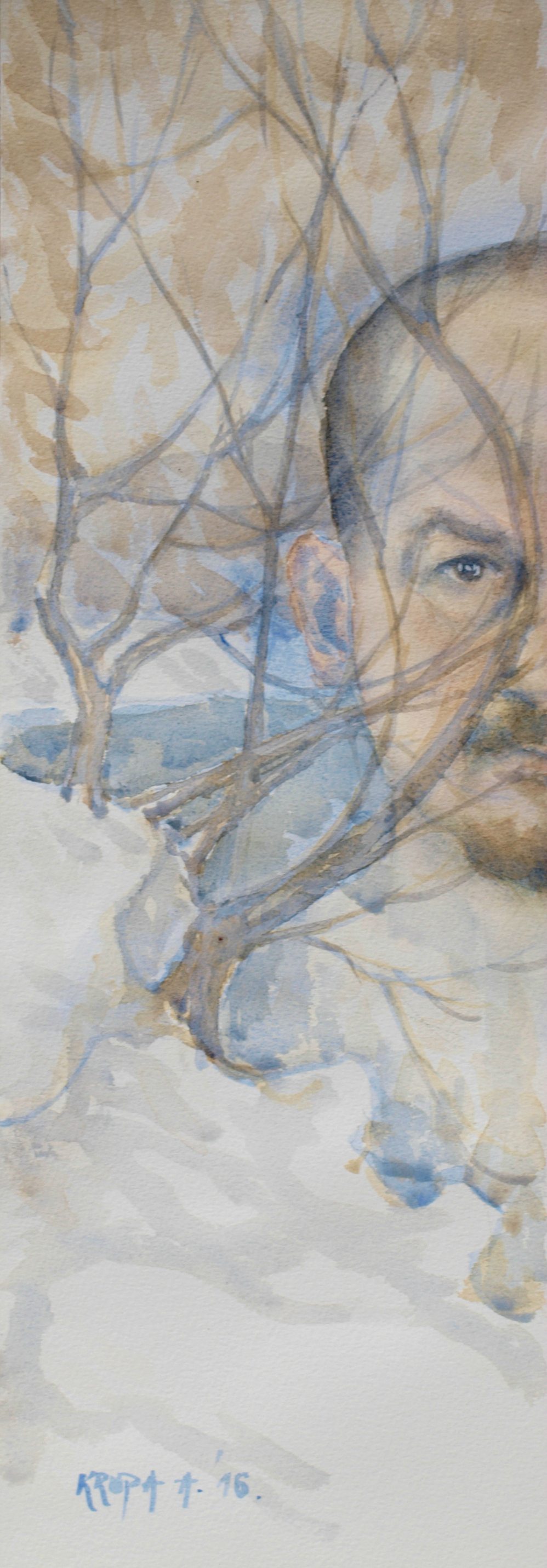This detailed, dreamlike painting features an intriguing overlay of imagery. On the right side of the composition is half of a man's face, exhibiting fair skin, a black eye, and a closely-cropped hairstyle with a receding hairline. His brown goatee and mustache add to his distinct appearance. Overlaying the man's visage is a depiction of light brown, swirling trees stretching upwards, adorned with lighter brown leaves and set against touches of blue tint, suggesting a wintry scene. The base of the painting hints at snow-covered ground. A largely indecipherable signature graces the bottom, ending with the number 16, while a faint blue watermark is noticeable in the bottom left corner. The overall effect merges both the man's face and the natural elements into a surreal, dual-layer composition.